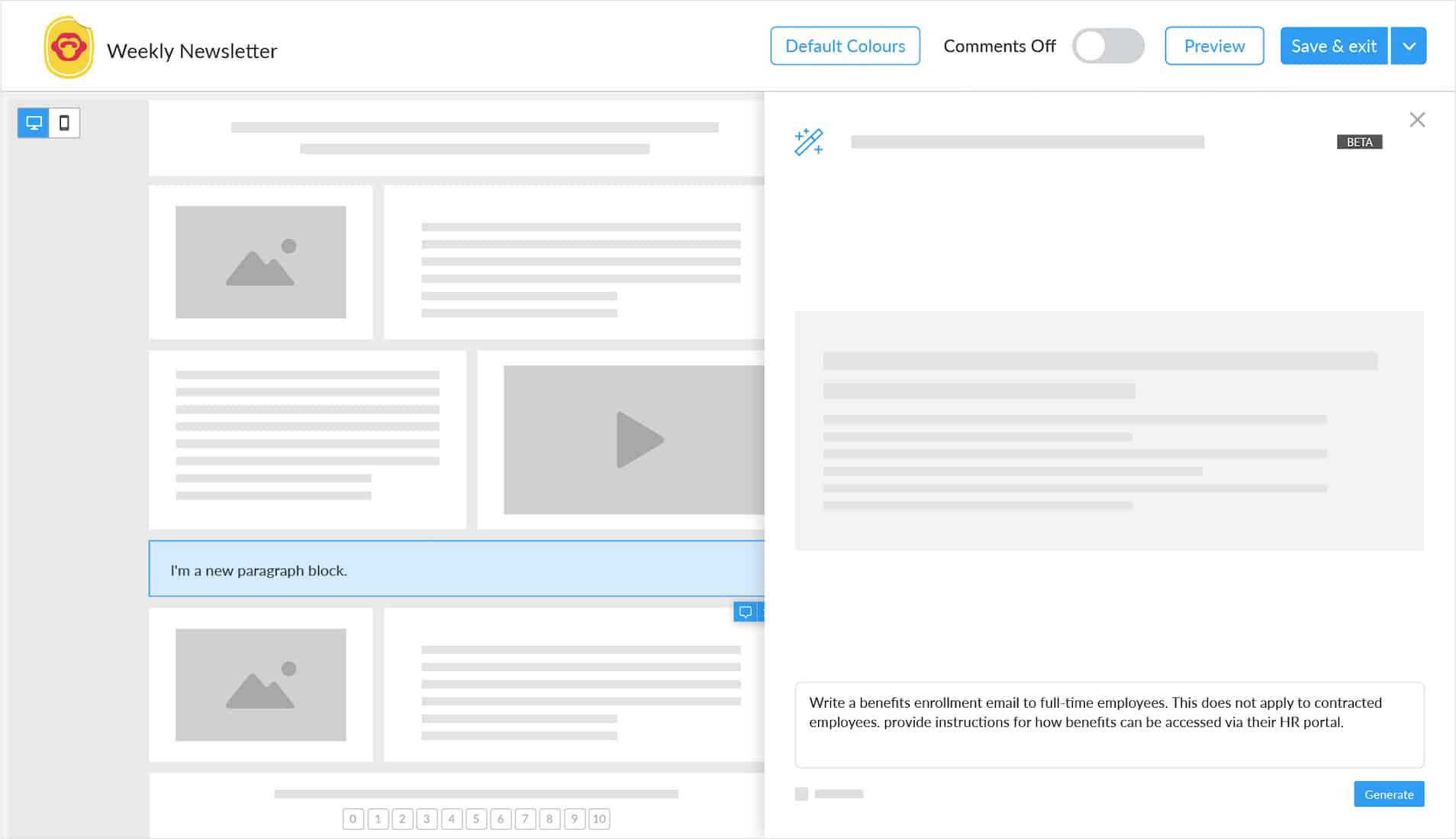In the upper left corner, a yellow circle contains the red outline of a monkey's face. Beside this, "Weekly Newsletter" appears in black text. Below, a large white box filled with plain gray lines is displayed. Adjacent to this is a light gray box with an image of a gray mountain inside it. This gray box includes a small gray arrow pointing to the right. Beneath this, a long blue box reads "I'm a new paragraph block."

On the right side, at the top, a blue box contains the words "default colors" next to "comments off," with a white circle adjacent to it and the word "gray" on the other side. Inside a blue square is the word "preview," and next to it, within another blue square, it says "save and exit." Below this, another long gray line appears, to the left of which is the outline of a blue pencil surrounded by some stars. In a small black box with tiny text, the letters "B-E-T-A" spell out "beta."